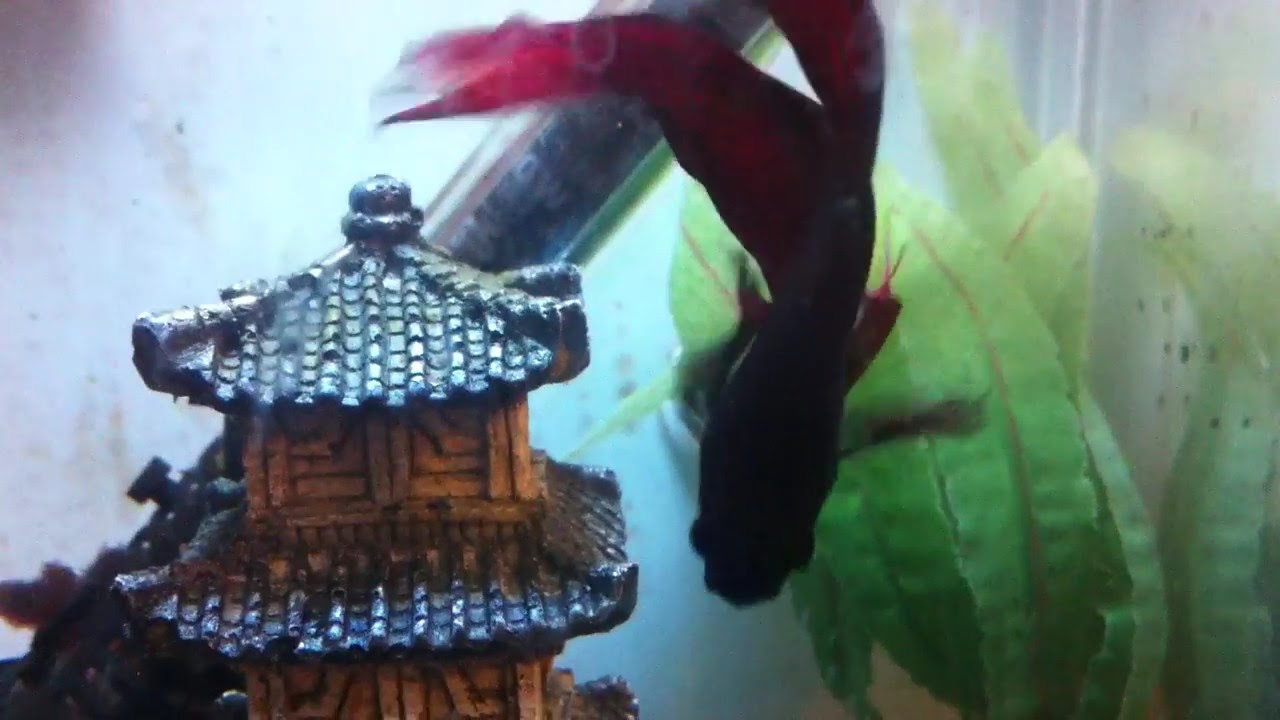The detailed image showcases the interior of a square fish aquarium. Dominating the forefront and center is a striking betta fish, predominantly black with a purplish shimmer. Its long, elegant fins and tails are vibrant shades of red. To the left side of the image, a decorative ceramic structure resembling a multi-storied pagoda with a shiny blue roof and brown wooden texture stands embedded in the gravel. Behind and to the right of the fish, a lush green plant with a red stem stretches upward, its wavy leaves adding a natural touch to the scene. The aquarium walls at the back and right side are speckled with various black and green dots, subtly framing the vibrant underwater scene. The water is clear, emphasizing the vivid colors and intricate details of this captivating aquatic setup.